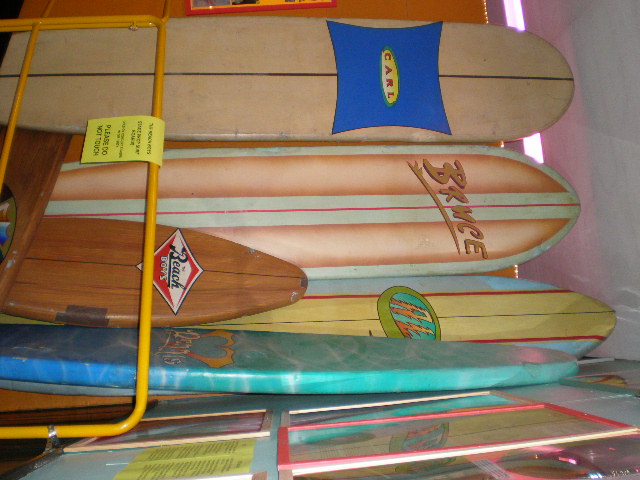The image shows a set of five surfboards standing vertically inside what appears to be a room, though the photograph is taken sideways, making the top of the picture appear on the right. Four of the surfboards are tall, while one is notably shorter. They are all positioned on a yellow dolly cart with an orange metal handle, suggesting that the cart is for moving these surfboards. 

The surfboard on the top (left side of the rotated image) is a beige color, featuring a black line running vertically with a blue square in the middle that says "Carl" in red lettering, bordered by yellow against a green background. To its right (next in sequence) is a white surfboard with a thin red line down the center, flanked by broader orange stripes. This one is labeled "Bruce" in brown letters. 

Continuing right, the next surfboard has blue edges with a central yellow stripe lined by red. A circle in the middle labels it "Al" in red and yellow lettering. The fourth surfboard has a light blue and teal color scheme, reminiscent of ocean waves, with white lines running through it. 

The fifth, shorter surfboard, positioned in front of the taller ones, is made of brown wood grain with a diamond-shaped logo that reads "Beach Boys." Additional details reveal a reflection through a window with pink curtains, various framed pictures hanging on the gray walls, and a yellow sign on the dolly cart which reads "Please do not touch."